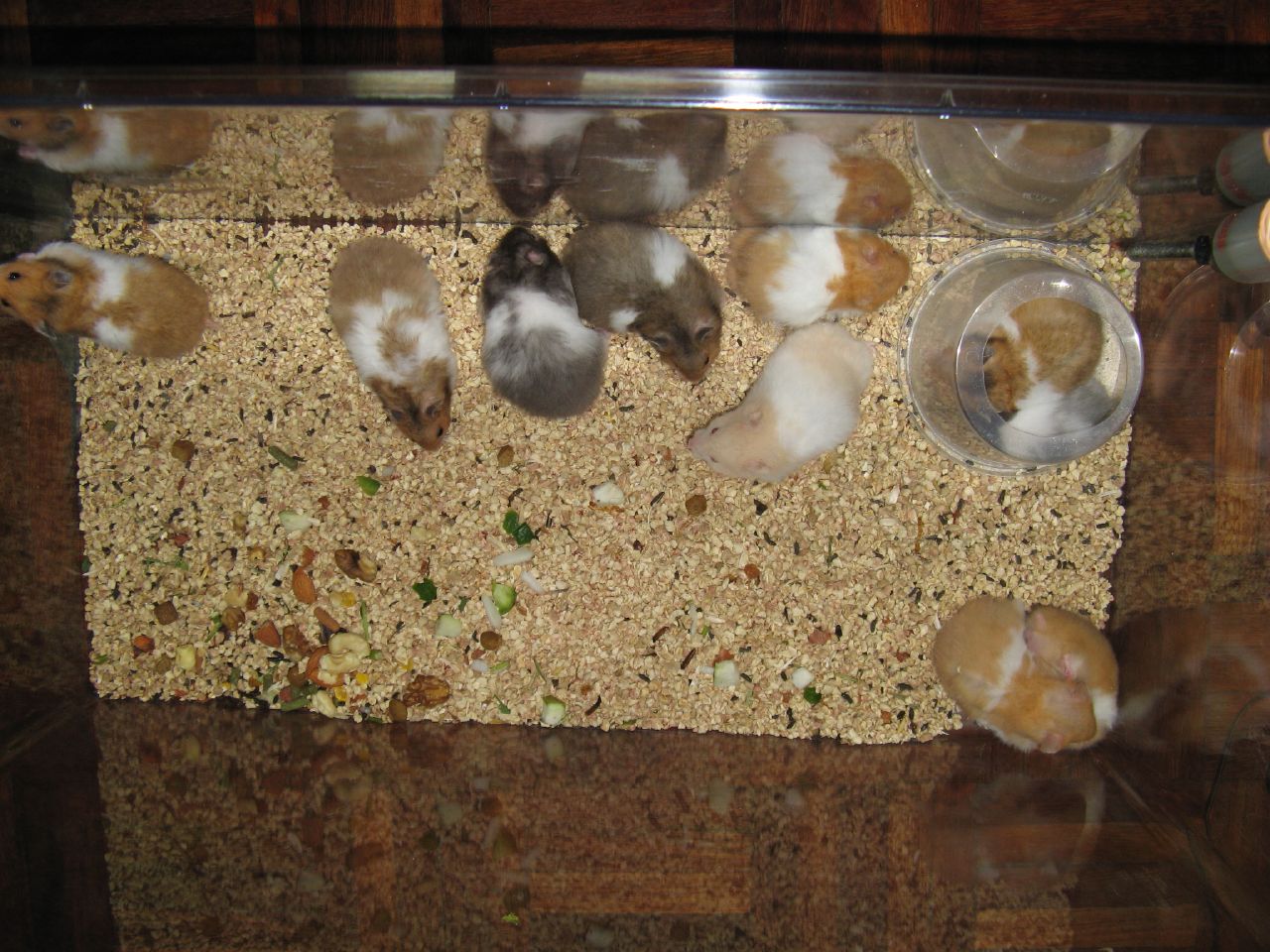In this bird's-eye view color photograph, eight hamsters with gray and brown fur are shown inside a glass cage. The bottom of the cage is lined with sand, which contains scattered small vegetables, primarily green, and what appears to be crushed nuts. Small brown shapes are visible among the mixed content. Six of the hamsters are gathered near the outer wall of the cage, while one hamster is positioned in the top right corner, isolated inside a small clear cup. The detailed mix of substrate and food highlights the hamsters' environment, suggesting a thoughtfully prepared enclosure for these small pets.